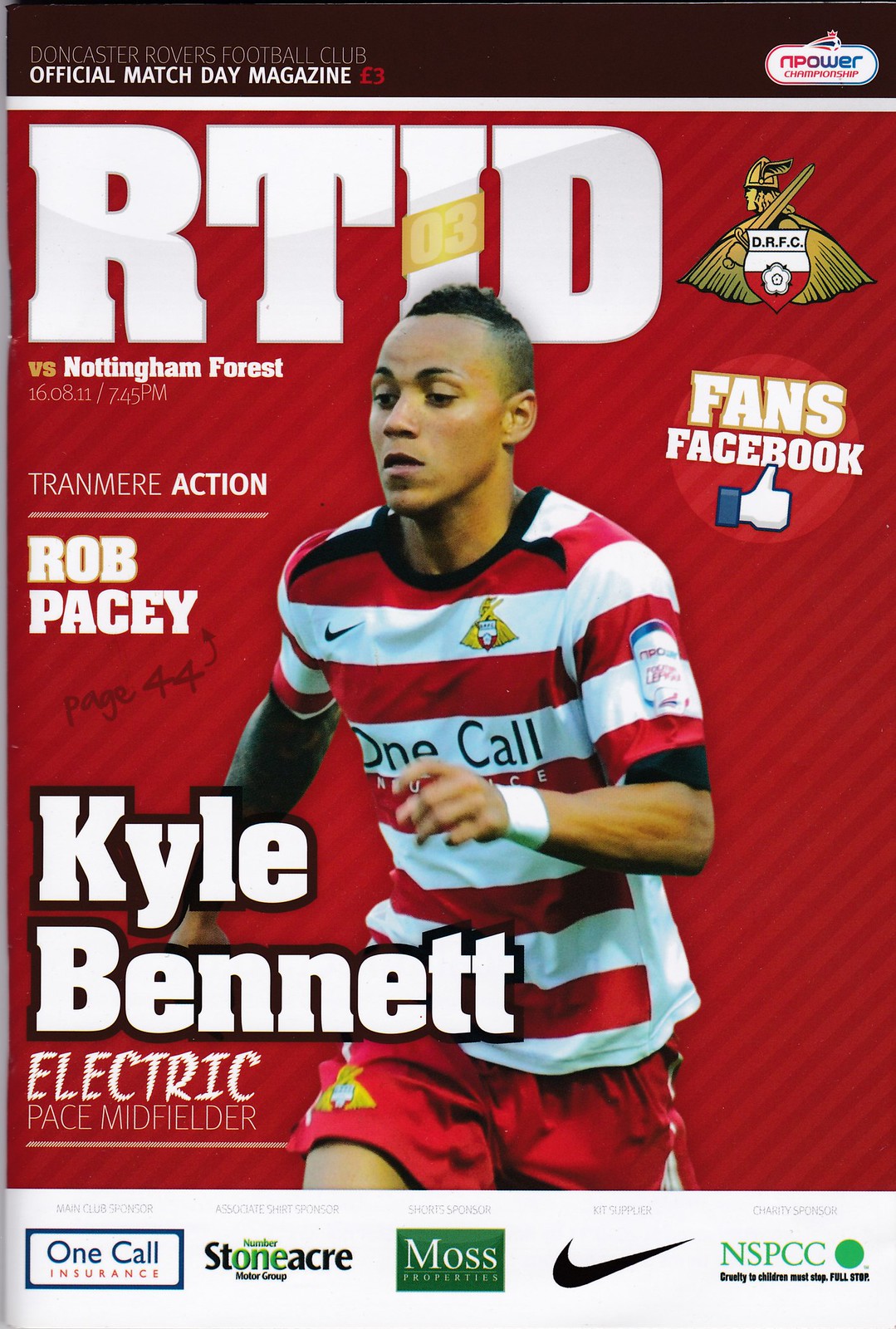The image is the cover of an official match day magazine for an English football club, featuring a prominent photograph of a player named Kyle Bennett. The cover has a distinct red background with white text. Kyle Bennett is pictured wearing a red and white striped shirt with a black check mark and a yellow mascot on the front, complemented by red shorts featuring the mascot design. He has a mohawk hairstyle and is sporting a white wristband. The magazine prominently displays text that reads “R.T.I.D.” in the upper left corner, and “One Call” along with various advertisements for One Call Insurance, Stoneacre, Moss, Adidas, and NSPCC. Below Kyle Bennett’s name, the text highlights his role as an "Electric Pace Midfielder." Additionally, it references an upcoming match against Nottingham Forest and topics like Tranmere Action and profiles on Rob Pacey and Kyle Bennett.